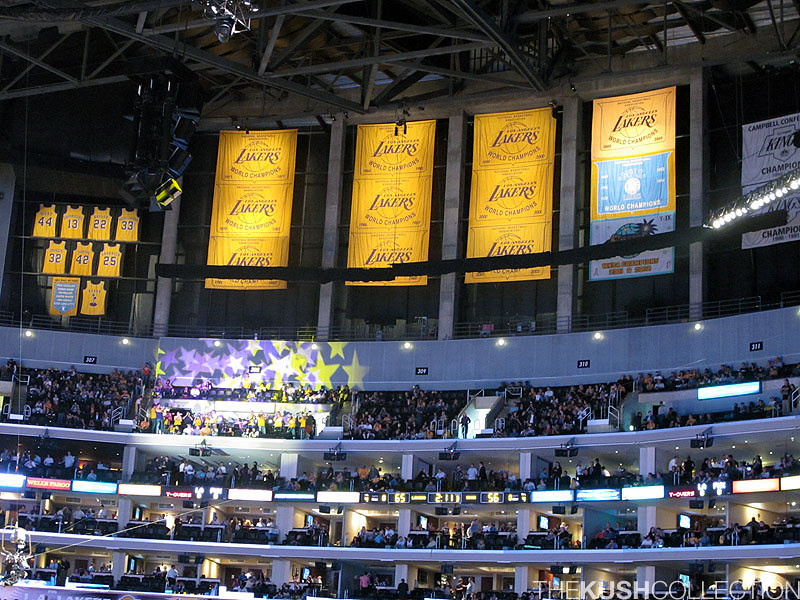This image captures the interior of a bustling basketball gymnasium for the Los Angeles Lakers. The top half of the image features a black wall adorned with five evenly spaced steel beams. On the left side, just below the ceiling, there is a glass case displaying yellow jerseys with purple numbers arranged in three levels. The top row has jerseys numbered 40, 44, 13, 22, and 33. The second row displays the numbers 32, 42, 25, and one obscured by a sign. To the right are three vertical columns of Lakers banners hanging from the rafters, each column containing three banners. The first column has three Lakers banners, the second has one Lakers banner at the top and a banner with blue and white writing below it, and the third column is partially obscured. 

In front of these banners are four rows of seating filled with spectators. The seating has a gray trim and is packed with people, making it difficult to see individual faces. There are also lights strung across various sections of the gymnasium, adding to the stadium's bright atmosphere. The scoreboard is positioned at the bottom center of the image, displaying the scores 65 and 56, and the time 2:11:3 in yellow digits.

The overall scene is vibrant and crowded, with fans eagerly watching possibly a game or a practice session, showcasing the rich heritage and the enthusiastic following of the Los Angeles Lakers.